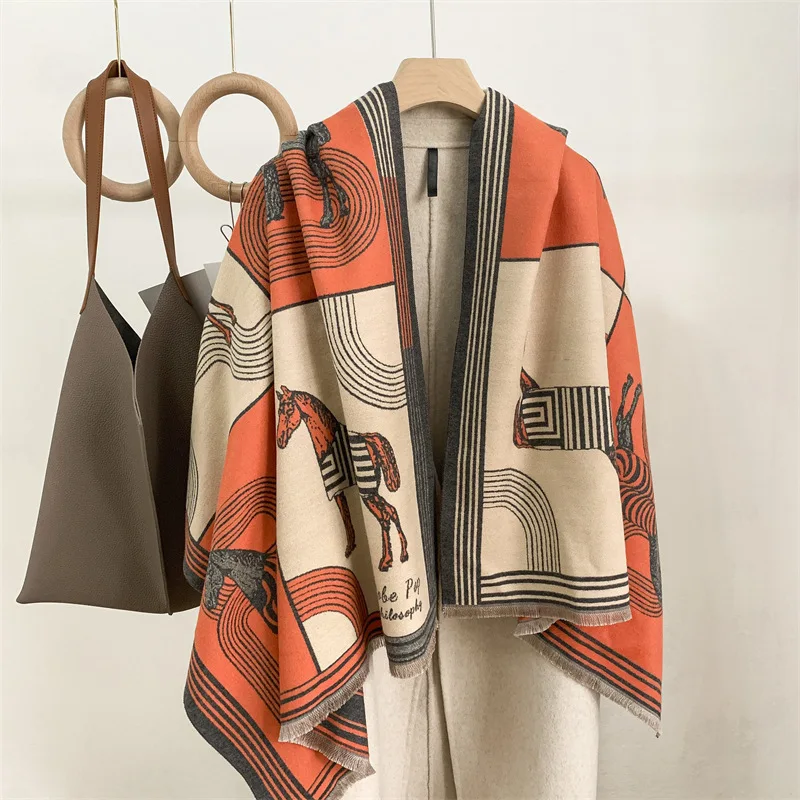The photograph captures a specialty clothing ensemble displayed in a manner reminiscent of a boutique setting, set against a flat, off-white backdrop. Central to the image, slightly biased to the right, is a handmade jacket draped over a wooden hanger. The jacket has a natural wool texture and is adorned with a vibrant shawl in shades of orange and beige. The shawl features various curved black artworks and prominently displays an orange horse embellished with a geometric pattern. Below the horse, there is some text, part of which reads "PA" and possibly "philosophy." Adjacent to the jacket, on the left, two wooden rings hang from the top. The ring on the far left suspends a stylish brown tote bag with a long brown handle, which adds a complementary touch to the display. The overall setting, combined with the detailed and artistic elements of the clothing, suggests a high-end, artisanal aesthetic.